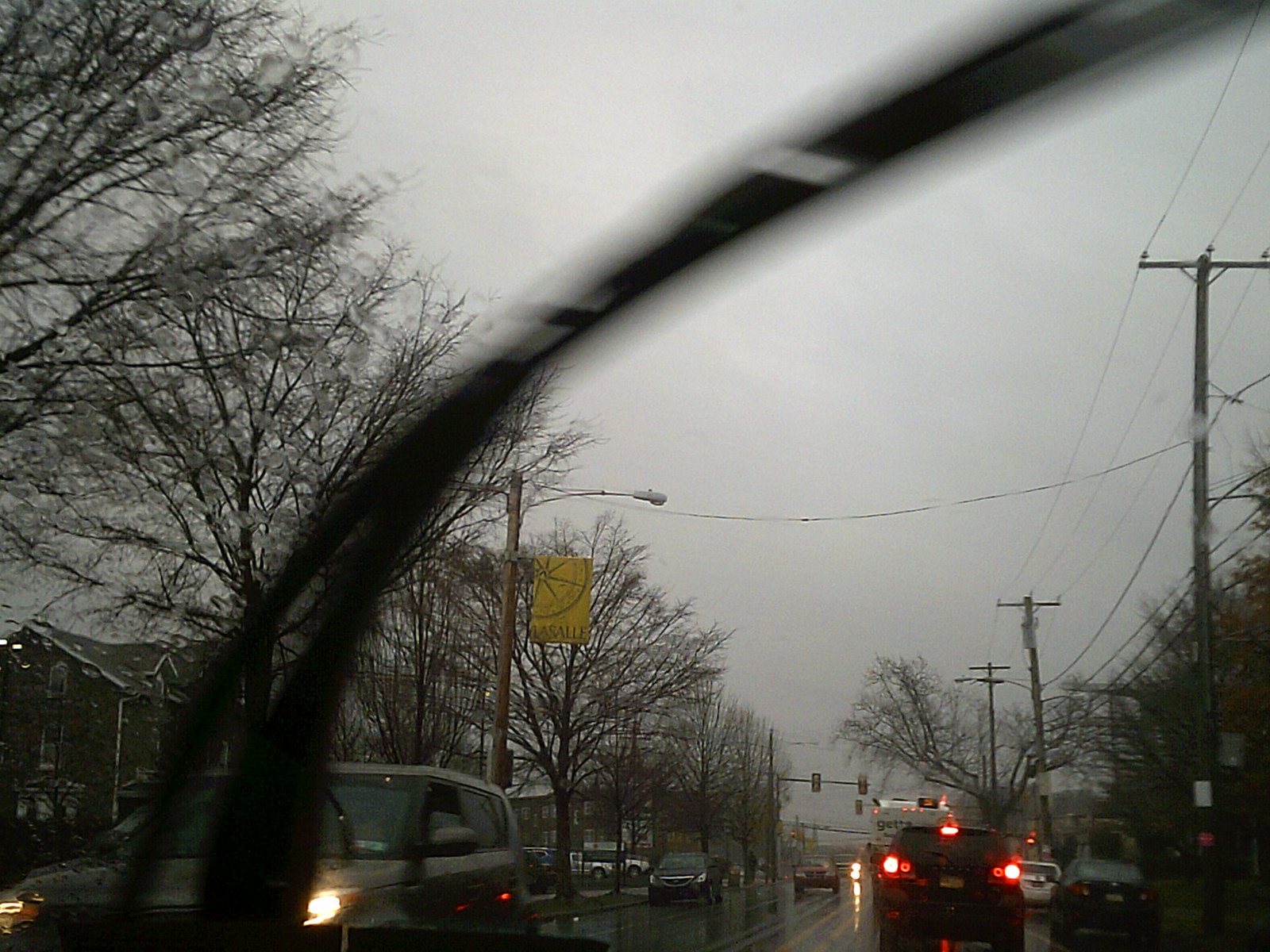A photograph taken through a car windshield depicts a dreary, overcast day. The sky is thickly blanketed with dark gray clouds, making it appear dim despite being daytime. The road ahead is framed by barren trees on both sides, their brown bark standing starkly against the gloomy backdrop, devoid of leaves. On the right side of the road, large electrical poles march alongside, connected by a web of wires. Additionally, a solitary street lamp is visible on the left side. Several vehicles are in view, their red brake lights glowing, suggesting a slow-moving or halted traffic. In the opposite lane, an approaching car has its headlights switched on. Cutting diagonally across the entire scene is a windshield wiper, caught mid-swipe at the moment the photograph was taken.